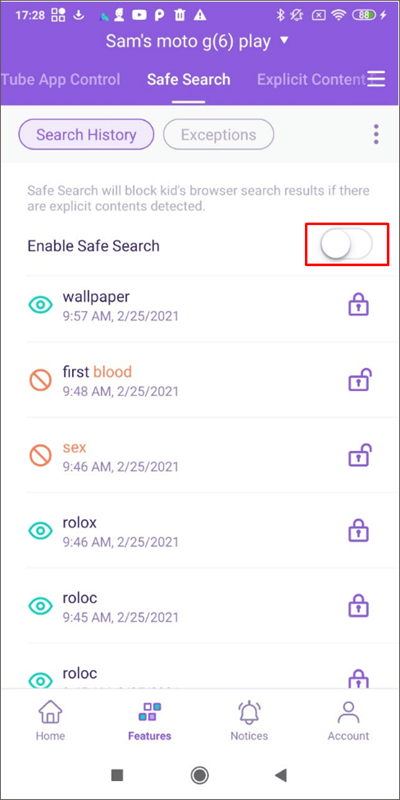Image Caption: 

The image displays a mobile interface against a bright purple background. At the top, the time is shown as 17:28. Below the time, the device name "Sam's Moto G (6)" is displayed in white text, followed by a small downward-pointing arrow.

Next, a battery icon is visible, indicating it is slightly below halfway charged with a green section on one side and the number "58" centered within the icon.

Below the battery icon, there is a section dedicated to "Tube App Control." The options listed include (from top to bottom):
1. "Safe Search" (underlined in white),
2. "Explicit Content" (with a purple background),
3. "Search History,"
4. An option labeled "Exceptions," which is on a white background outlined in gray.

A description in black text explains that enabling "Safe Search" will block explicit content from children's browser search results. The "Enable Safe Search" option is depicted with a toggle switch inside a red box; the switch is currently in the off position, toggled to the left.

Following this section, there is another segment titled "Wallpaper," with an image of a blue circle beside it. Below this, timestamps and titles are listed as follows:
- At 9:57 AM on 2-25-2021, "First Blood" is marked in orange,
- At 9:48 AM, "Sex" is marked with an orange circle crossed out,
- At 9:46 AM, "Rolox" (spelled R-O-L-O-X) appears with a green circle beside it,
- Another item listed as "Roloc" (spelled R-O-L-O-C).

This concludes the visible information from the interface image.